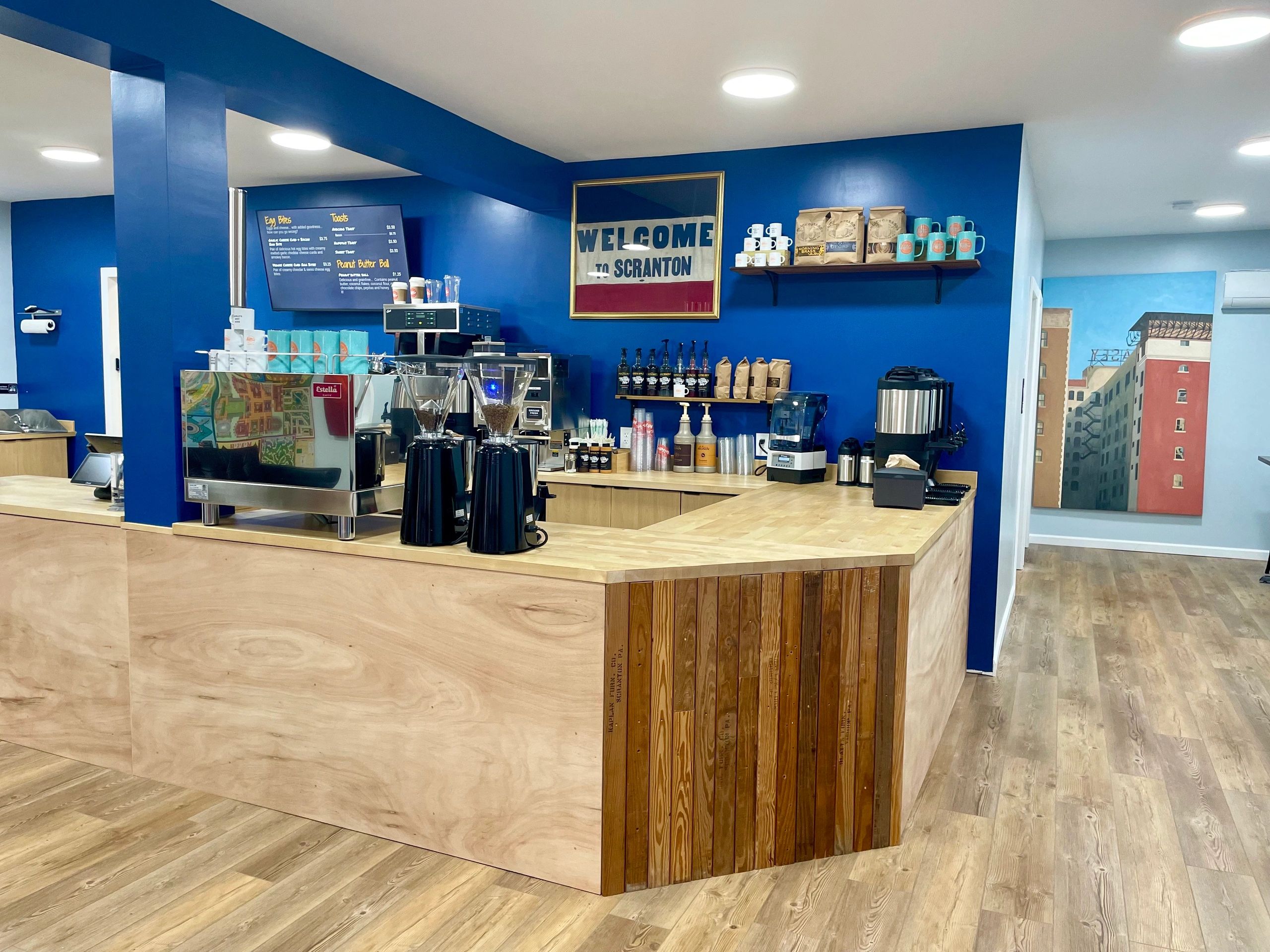In this image, a quaint café or coffee shop setting is depicted. The foreground features dark blue walls that contrast with the light blue walls in the background. Prominently displayed in the background is a large poster showcasing a red brick building surrounded by lighter-colored buildings. The café has a charming wooden floor, adding warmth to the atmosphere. A spacious wooden counter, predominantly light-colored with a distinct darker brown wood at the corner, stands at the center. Atop the counter are various coffee makers and drink machines, emphasizing the shop's beverage offering. A patriotic sign reading "Welcome to Scranton" in bold blue letters on a red, white, and blue background adds a local touch. Additionally, a blue menu with yellow lettering hangs proudly in the background, completing the cozy and inviting ambiance of the café.